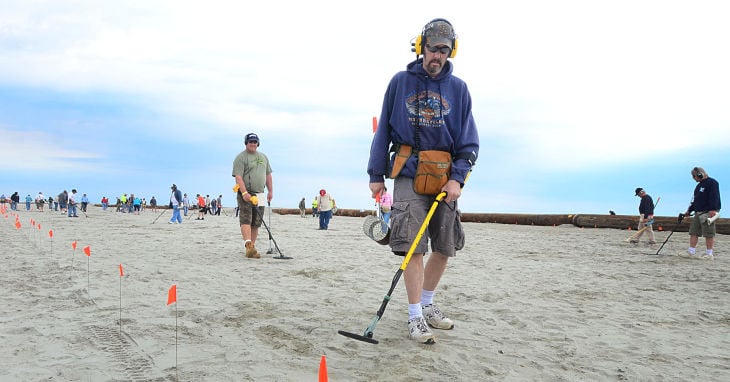This image captures a group of men methodically scanning a white to grayish sandy beach with metal detectors on a somewhat cloudy day. The sky is predominantly covered with light, fluffy clouds, primarily white with a tinge of blue near the lower atmosphere. In the background, a pipe runs parallel to the shoreline, and numerous small orange flags mark off a designated area on the beach.

In the forefront stands a Caucasian male, sporting dark sunglasses and a goatee. He wears a gray cap with yellow-coupled headphones strapped over his ears. His attire includes a navy blue hoodie with an image on the front, gray khaki cargo shorts, white running shoes, and white socks. He carries a metal detector with a yellow handle that transitions to black towards the bottom and ends with a flat, round piece used for scanning the sand. Attached to his waist is an orange pouch, presumably for collecting found items, and he holds a sifting cup.

Behind him, another man in a black ball cap, green top, and grayish khaki pants with brown boots mirrors his actions, also wielding a metal detector. In the distance, several other individuals similarly clad in hoodies, cargo shorts, and jeans, concentrate on their metal detection work, all contained within the area marked by the orange flags. The scene emphasizes a shared intent among the men to unearth metallic fragments from the beach.